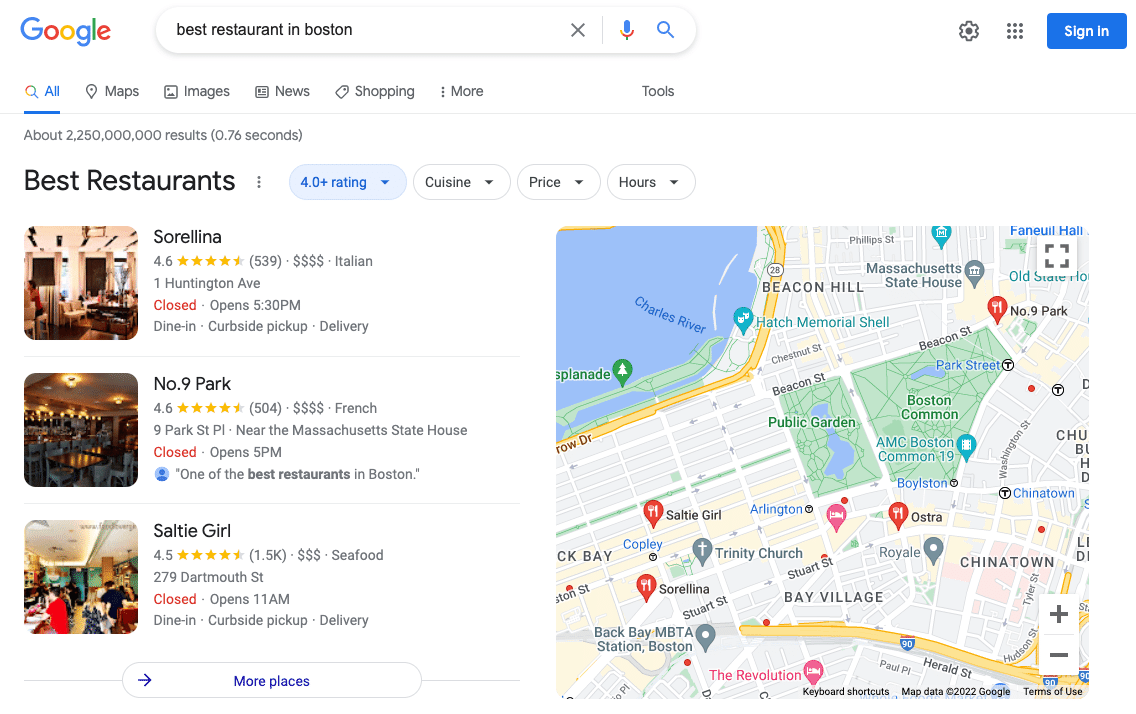The image is a horizontally rectangular screenshot of a Google search page against a white background. In the upper left corner, the colorful Google logo is prominently displayed next to the search field where the phrase "Best Restaurant in Boston" is typed. Below the search bar, navigation tabs for “All,” “Maps,” “Images,” “News,” “Shopping,” and “More” are visible, guiding users toward different types of search results. 

Directly beneath these tabs, the header "Best Restaurants" is in bold, accompanied by a drop-down filter menu set to "4+ rating." Other filter buttons, including "Cuisine," "Price," and "Hours," remain unselected. The main content area features three vertical listings for highly-rated restaurants, displayed with small images showing the interiors. The listed restaurants are: Sorrelina, Number 9 Park, and Salty Girl. 

On the right side of the page, there is a large square map dotted with location markers, offering a visual representation of the restaurants' positions within Boston.